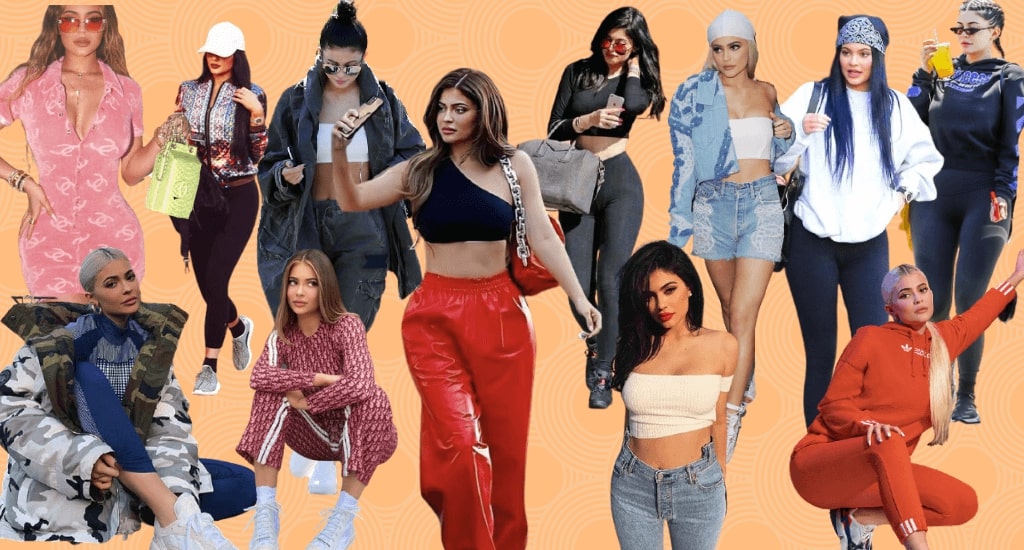A dynamic collage featuring an array of women, possibly the same person or different people, is set against a light tangerine background adorned with faint white circular designs. Central to the image is a striking woman wearing a black halter top that exposes her midriff, paired with shiny red pants and a chain over her right shoulder. She holds a smartphone up to her face, her long black hair draping over her shoulder. To the lower right, a woman in a tight white top and blue jeans, displaying her midriff, stands out with dark black hair and red lips. Beside her, a woman in an orange jumpsuit kneels, her blonde ponytail cascading almost to her stomach. In the far bottom left, a woman sits in a black and white camouflage coat with hints of green, beneath another woman in a pink dress that showcases her cleavage and accessorized with orange sunglasses. The image is a celebration of diverse, trendy fashion and hairstyles, reminiscent of celebrity magazine cutouts, featuring between 10 to 15 distinctly stylish figures.